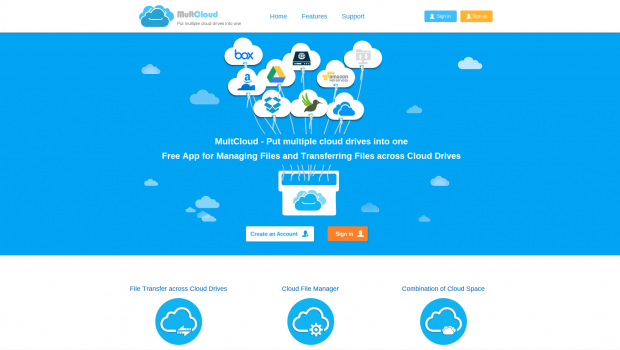This image is a screenshot of a website featuring a dual-tone design with a white header and a predominantly sky-blue background. 

At the top left of the header, the text "Multi Cloud" is prominently displayed, with "Multi" in gray font and "Cloud" in sky blue. Adjacent to this, the company logo features a blue cloud with two lighter blue clouds on either side. 

The top menu, written in light blue font, includes three options: "Home," "Features," and "Support." Towards the right of the header, there are two rectangular buttons. One is blue with the text "Sign In" accompanied by an account icon, and the other is gold with the text "Sign Up."

In the main section of the website, the background is a beautiful shade of sky blue, adorned with small white cloud illustrations. Within these clouds are icons for various services such as Dropbox and Google Drive. 

Centrally positioned on the page is a headline in white font that reads, "Multi Cloud: Put multiple cloud drives into one free app for managing files and transferring files across cloud drives." 

Beneath this, there is a small illustration of the Multi Cloud logo on what appears to be a white box.

At the bottom of the page, the background shifts to white and features three blue circles. Each circle contains a simple white outline drawing of a cloud. The headings for these sections, from left to right, are: "File Transfer Across Cloud Drives," "Cloud File Manager," and "Continuation of Cloud Space."